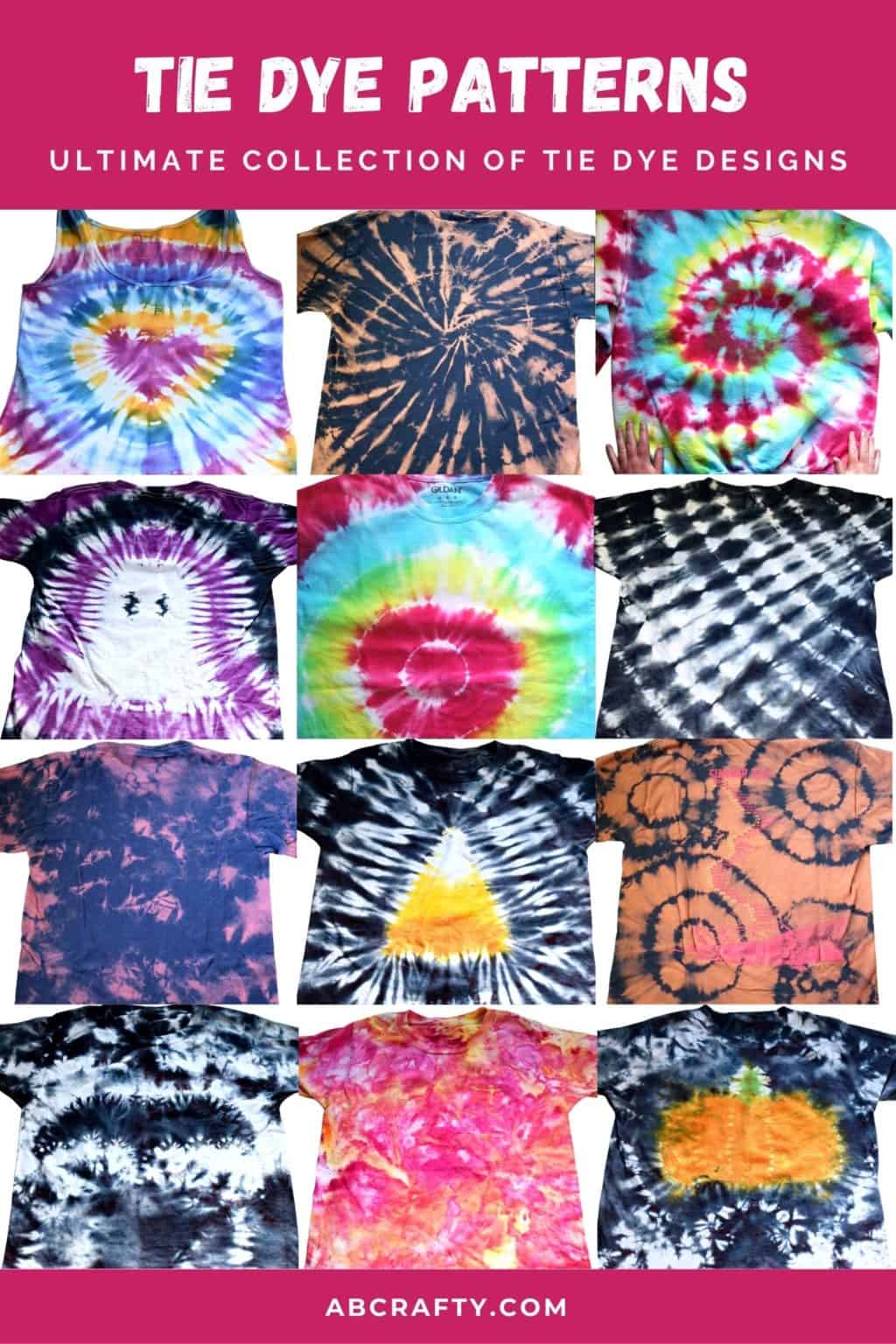The advertisement image showcases a vibrant array of twelve tie-dye shirts, meticulously organized into four rows of three. At the top of the image, bold white text on a burgundy background declares "Tie-Dye Patterns, Ultimate Collection of Tie-Dye Designs" in all caps. At the bottom, a matching burgundy strip features the URL "ABCrafty.com" in white text. The shirts exhibit a diverse palette of tie-dye designs and colors, including a black and white shirt with an acorn design, a striking rainbow swirl, a shirt in shades of gold, green, and teal blue, and a unique pattern with black and gold colors. One shirt even features a pumpkin design, while another showcases a distinctive mix of brown with black circles and a splash of pink. Each shirt is uniquely colored, further illustrating the vast possibilities of tie-dye patterns available from ABCrafty.